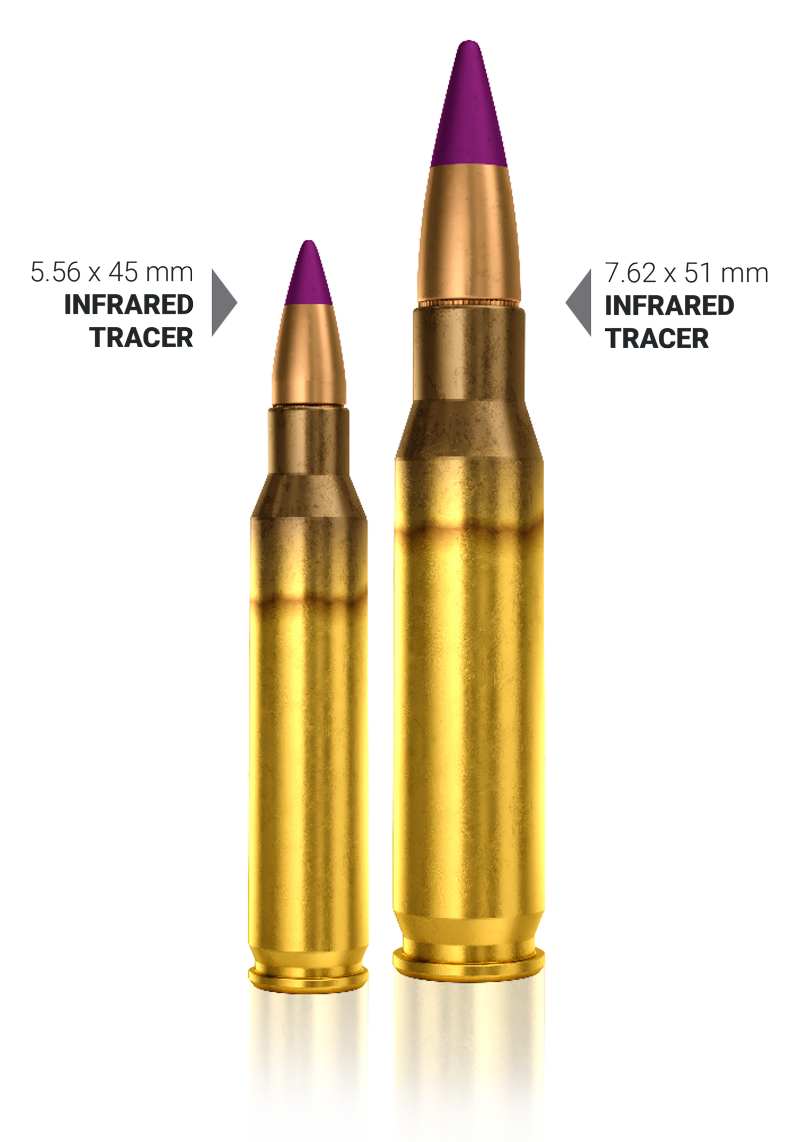The image depicts a close-up of two rifle bullets against a completely white background. On the left side, a golden, slender bullet labeled "5.56x45mm infrared tracer" features a purple tip and has a grey arrow pointing to it. This bullet is long and tapers to a pointed top. To the right of it, a slightly larger and thicker golden bullet also with a purple tip is labeled "7.62x51mm infrared tracer," and similarly, a grey arrow points to this bullet. Both bullets have visible labels in black font next to them, detailing their size and function as infrared tracers, designed to help shooters track the path of their shots.